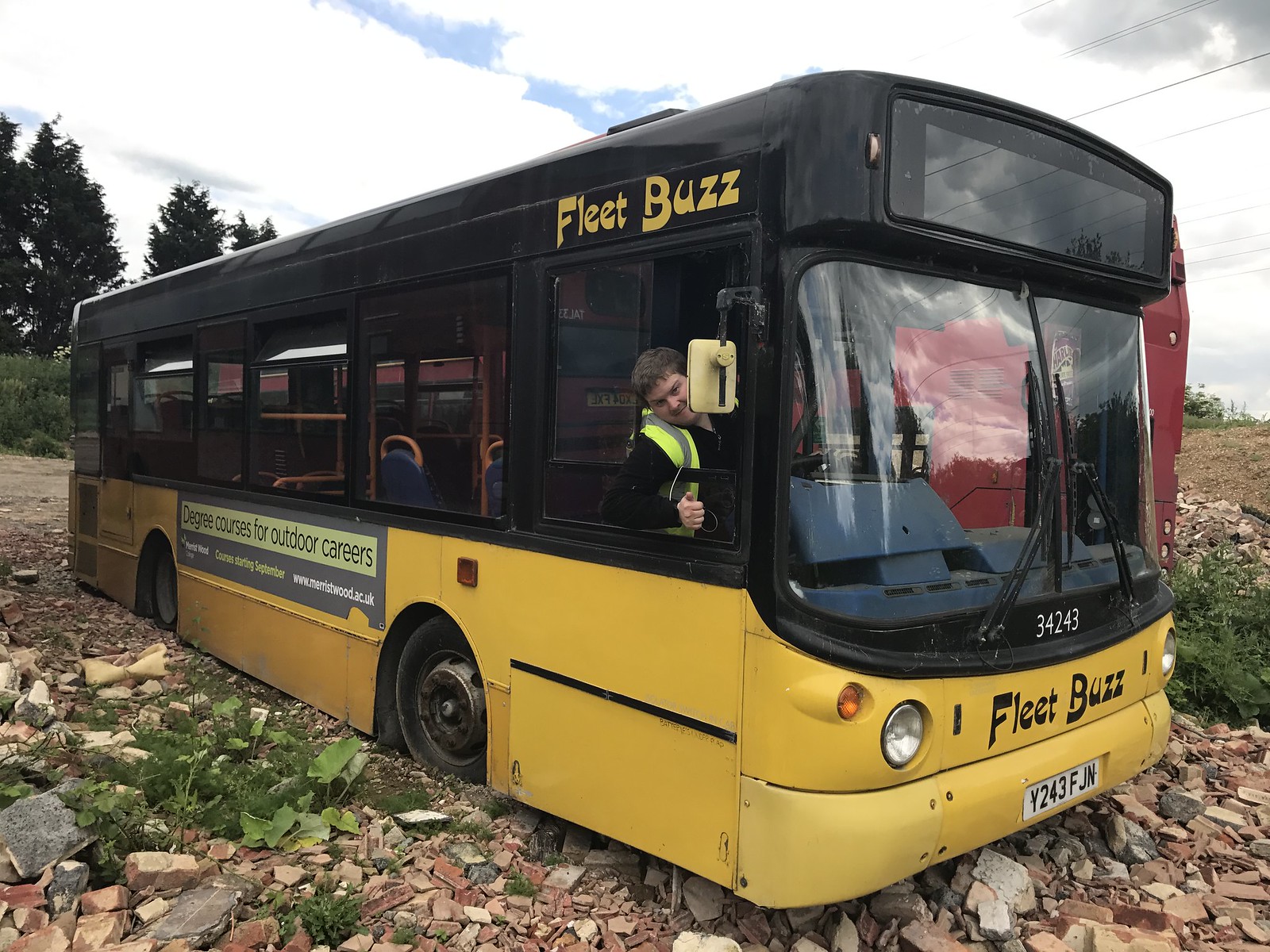The photograph depicts a colorful bus on a rocky dirt ground, seemingly situated in a rural area. The bus has a distinctive paint scheme with a black upper half and a bright yellow lower half. It's positioned such that both the right side and the front of the bus are visible. Across the front of the bus, and above the driver's window on the right side, the text "Fleet Buzz" is prominently displayed. 

The bus appears to be in a state of disrepair, as its tires are flat and the bottom of the bus is nearly in contact with the uneven ground, which is littered with rocks and other debris. In the background, to the left side of the bus, there is a hint of a dirt road and some distant trees. To the right, there is an expanse of grassy and dirt field.

A man is leaning out of the window on the right side of the bus, beneath the "Fleet Buzz" text. He is wearing a yellow safety vest over a dark shirt and has medium-length brown hair. His hand is raised in front of him, and he appears to be smiling. Beside him, the rearview mirror is visible. 

Notable details on the bus include a partially visible advertisement on the yellow top panel, and the numbers "34243" in white on the front. There's an additional "Fleet Buzz" marking below this, along with a license plate reading "Y243 FJN." An inscription on the side of the bus promotes "Degree courses for outdoor careers," though some of the text is obscured and difficult to decipher.